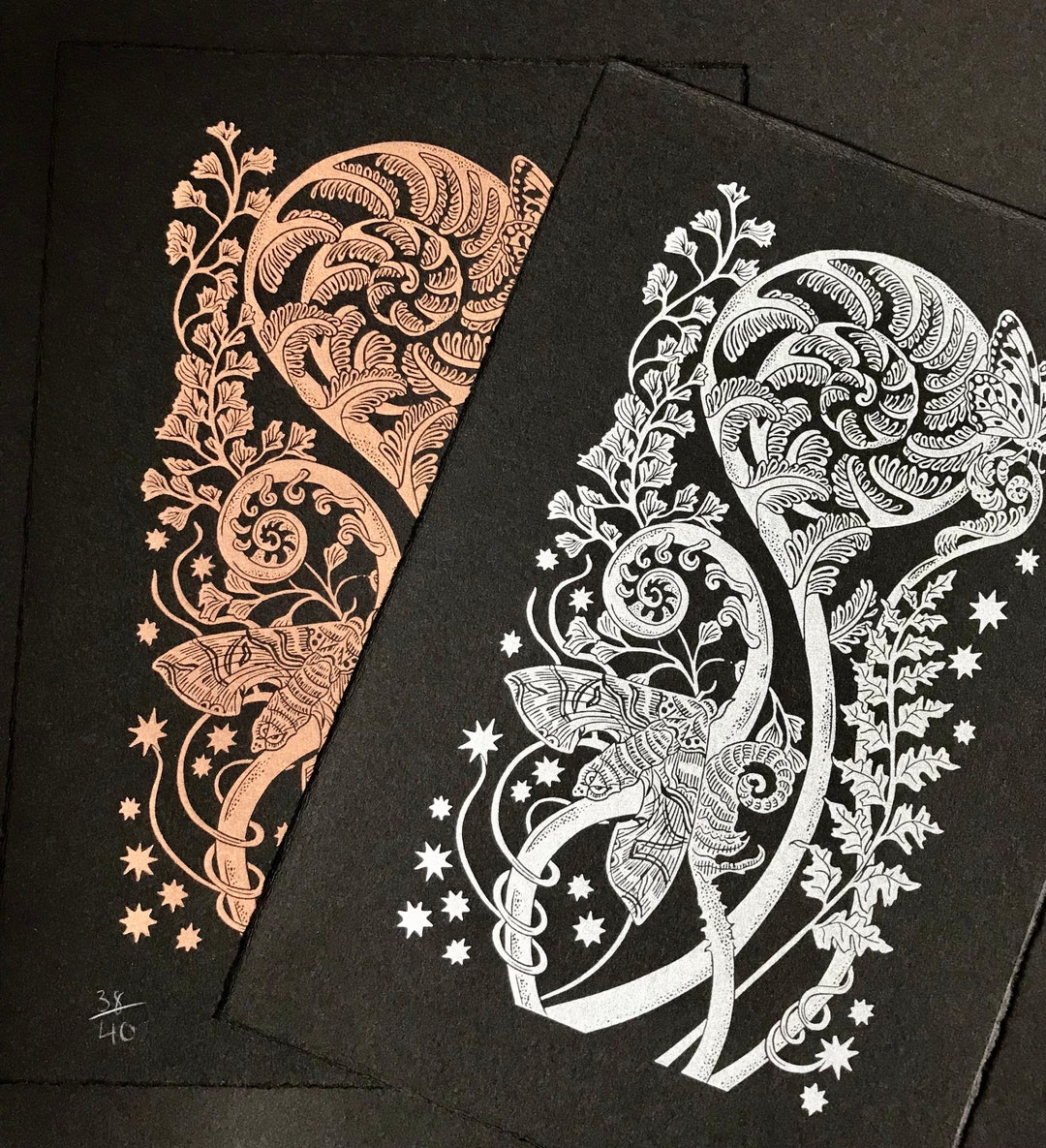The image features two intricate art prints displayed on a black backdrop. Both prints are identical in design but differ in color; one is rendered in white, while the other is a copper or peach tone. Each print showcases a detailed composition of moths and flowers intertwined with various vines. The vines are adorned with both large and small leaves that curl and stretch out in different directions. Scattered among the vines are numerous stars, creating a celestial ambiance. Notably, the print details are inscribed at the bottom left, with the white print marked as 39 out of 40 and the copper print as 38 out of 40. The overall aesthetic, characterized by its elaborate and delicate design, imparts a sense of beauty and wonder.